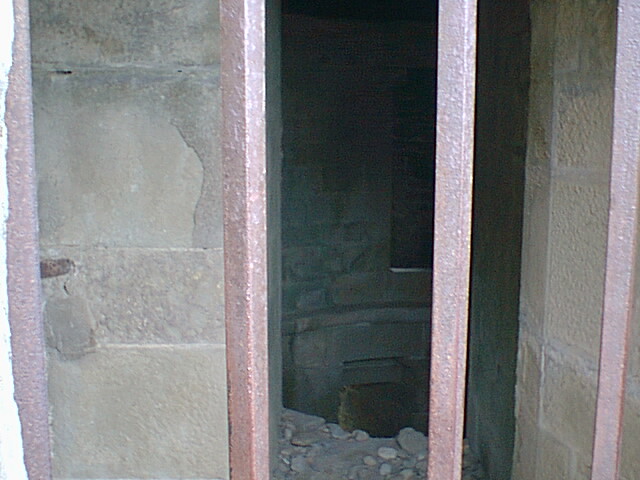The photograph captures the interior of an abandoned, dilapidated building seen through a doorway or similar opening, possibly hinting at a construction site. The scene is shrouded in darkness, with white light piercing in from the location of the camera, casting the rest of the room into shadow. The viewer's gaze is directed through red metal bars that block off a pathway, suggesting restricted access to prevent further exploration. Scattered broken concrete and rocks litter the pathway leading to a deeper, shadowy space where the floor appears to have collapsed or descends into a well-like area. The opposing wall, constructed from cinder blocks, dominates the scene with its tan, stone-like appearance. A vertically long, rectangular window with a curved arch at the top is set into this wall, contributing to the eerie, abandoned ambiance.